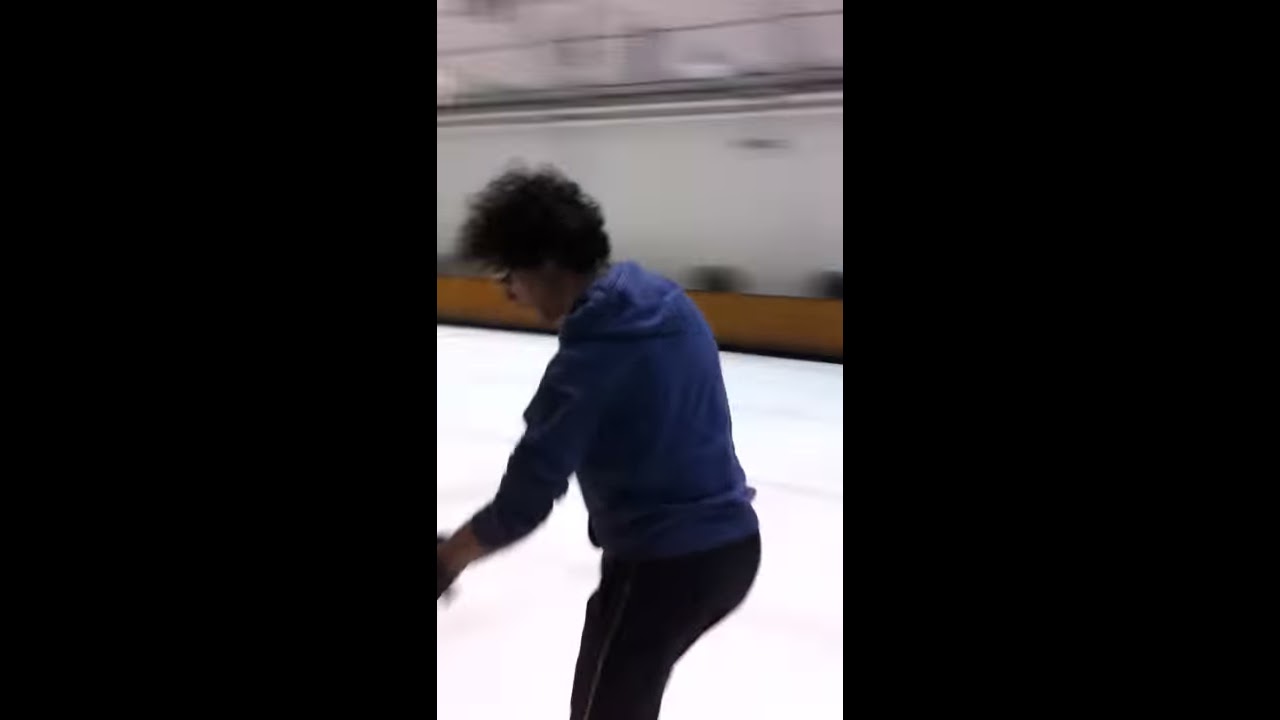A blurry portrait-oriented photograph captures a young boy with glasses and curly black hair ice skating in an indoor rink. He wears a navy blue hoodie and dark pants while standing on a white ice surface. The image prominently features him in a skating motion, though his feet are not visible, only his legs up to his knees. The rink is bordered by a round, yellow edge, and there's a white wall in the background, framed by two vertical black strips on either side of the image. The man appears focused on his movements, suggesting he is engrossed in perfecting his skating maneuvers. The surrounding colors blend into a mix of blues, blacks, whites, and browns due to the motion blur, emphasizing the dynamic nature of his activity.